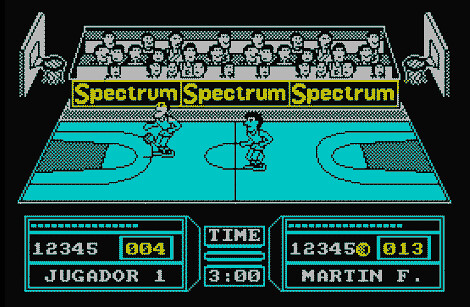This image showcases a retro-style basketball video game reminiscent of classic Game Boy graphics. The scene features a teal-colored court with two basketball hoops on either end, rendered in a minimalist black-and-white palette. Belonging to an era of pixel art, the stands are sparsely populated with spectators, adding to the nostalgic feel. The game is in progress with two players: Yugador, who has scored 4 points, and Martin F., leading with 13 points. The timer, positioned prominently on the screen, displays 3, indicating that the game is far from over.